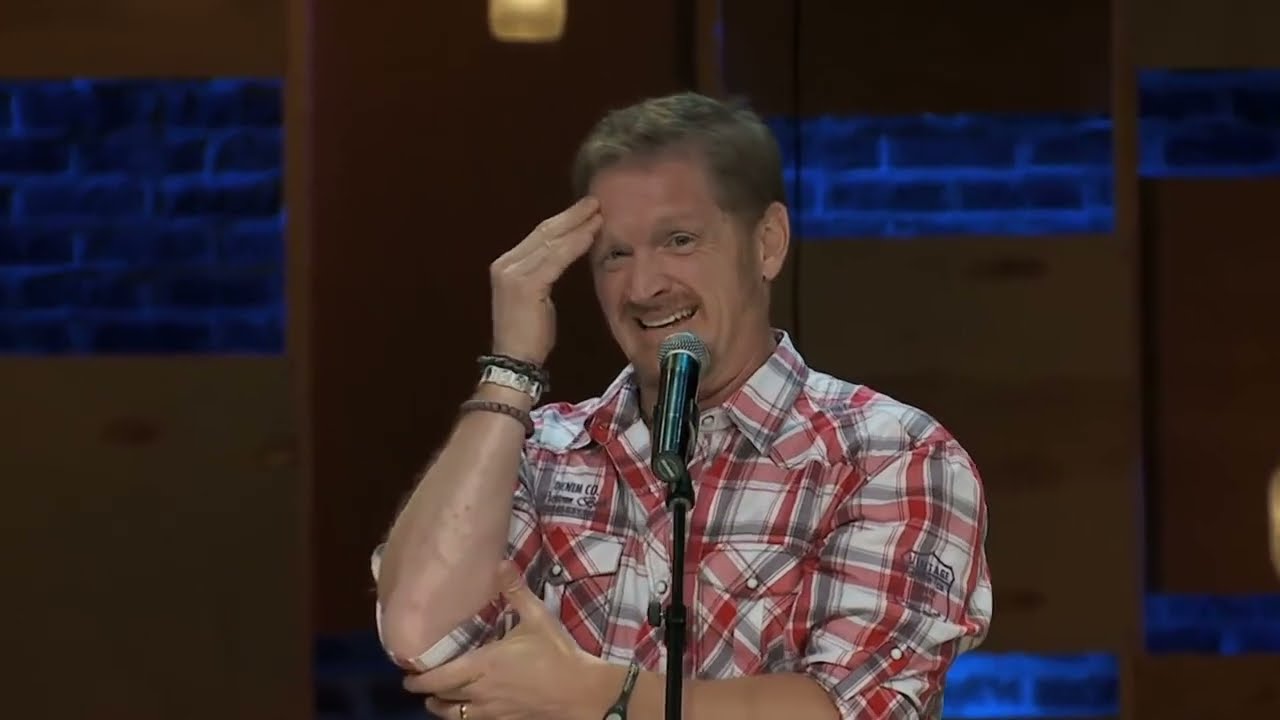The image features a man of lighter skin complexion with short light brown hair and a brown mustache, standing in front of a microphone on a stand, suggesting he might be performing stand-up comedy or speaking in public. He wears a red, white, and gray plaid patterned flannel shirt, with the sleeves rolled up to his elbows. His right hand is bent at the elbow, with his fingers resting on his forehead, conveying a mixture of stress and embarrassment, yet he is smiling. His left hand supports his right elbow, and on his left wrist, he wears a watch or bracelet and a wedding ring on his left ring finger. His right wrist is adorned with three bracelets – two black and one silver. The background consists of brown wooden panels with sporadic blue bricks on the left side and two panels featuring blue bricks at the top and bottom sections.